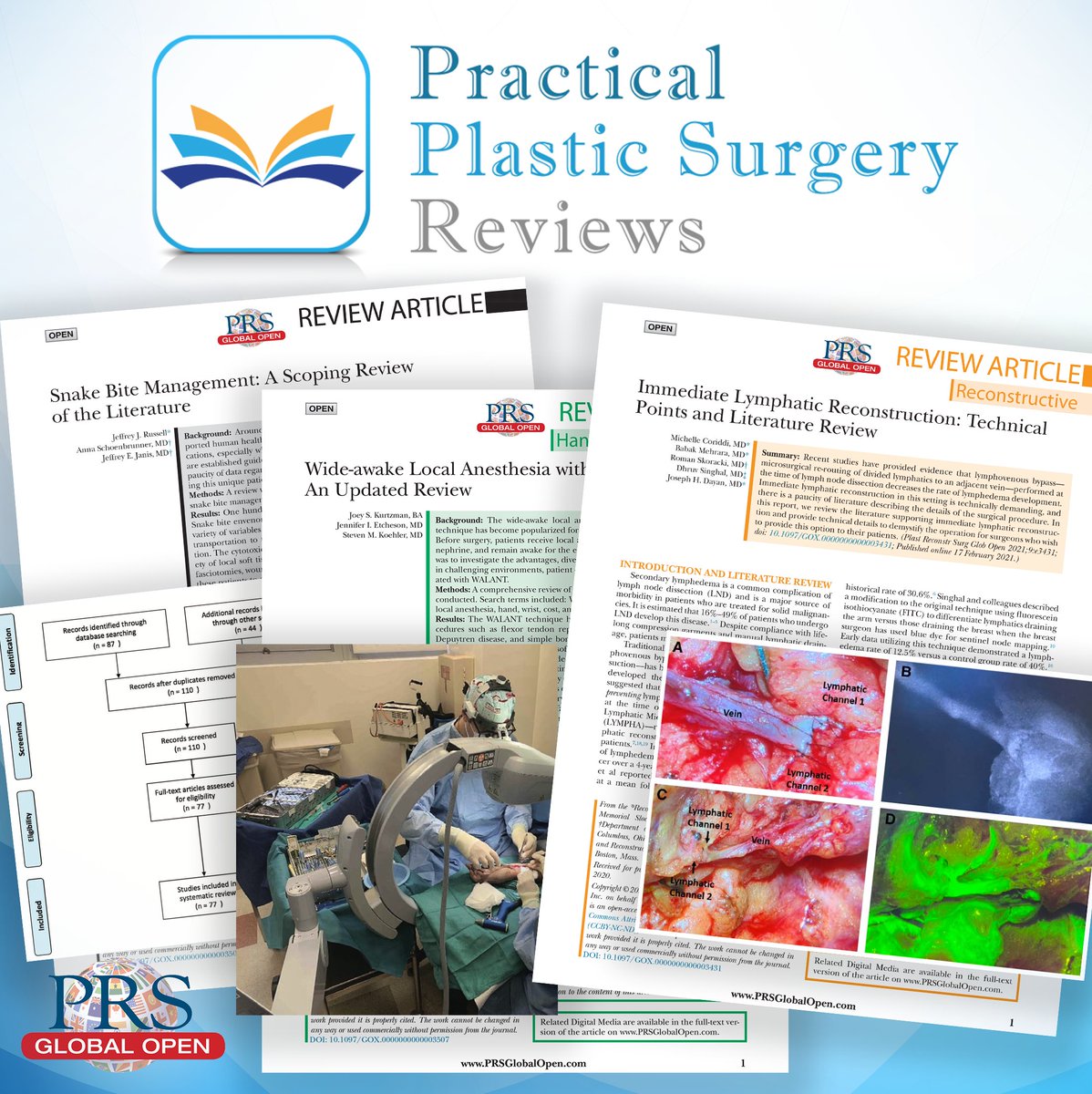The image prominently features the title "Practical Plastic Surgery Reviews" in teal, light blue, and gray text. Accompanied by a logo resembling an open book with a blue square outline, the pages of the book are colored yellow, blue, and dark blue, symbolizing the emblem of the publication. Below the logo, "PRS Global Open" is displayed, emphasizing its connection to the field. 

To the left, there's a section labeled "Review Article," featuring detailed topics such as "Snakebite Management: A Scoping Review of the Literature," which provides a comprehensive overview of snakebite treatments. Another article is titled "Wide Awake Local Anesthesia: An Updated Review," covering advancements in anesthetic techniques. The third article, "Immediate Lymphatic Reconstruction: Technical Points and Literature Review," delves into reconstructive surgical methods focusing on lymphatic systems, illustrated by four detailed images labeled A, B, C, and D. Image C shows some blood, while images B and D highlight structures in blue and green, respectively. The background of the image remains predominantly white, giving a clean, professional appearance.